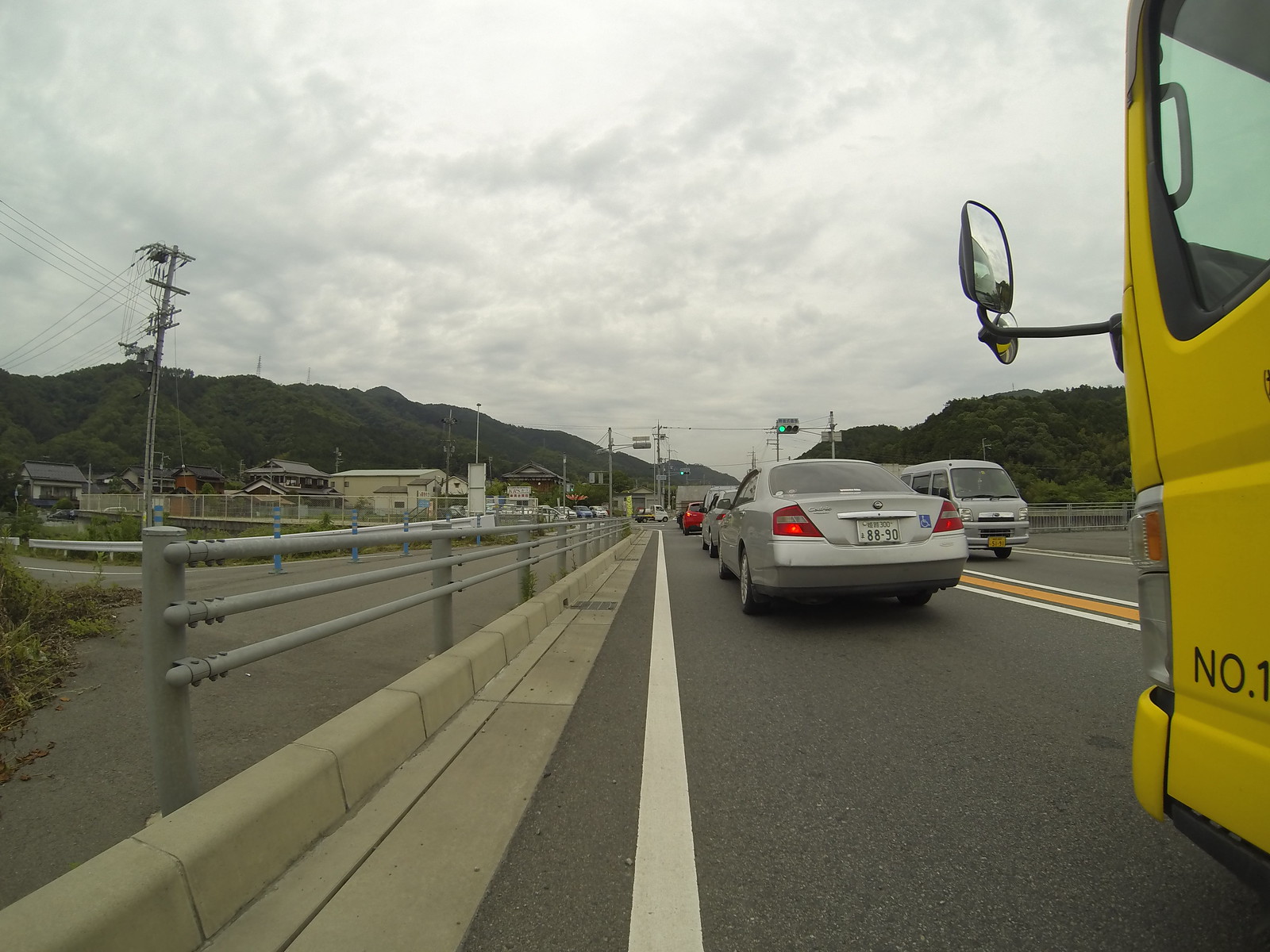In this rectangular, horizontally oriented vintage-style photograph with muted colors, we see a busy road scene that appears to be situated in a European country or an island outside the United States, as indicated by the reversed traffic lanes. The road features one lane in each direction. A silver sedan with a white license plate is traveling away from us, and in the lower right corner, a yellow vehicle, possibly a bus or truck, is partially visible. The paved road is marked with yellow and white lines and is flanked by metal fences or gates on both sides.

In the far left portion of the image, a range of mountains serves as a picturesque backdrop to a line of buildings. These buildings, some of which are likely homes and others possibly businesses, create a quaint, distant landscape. There is noticeable traffic on the road and additional vehicles parked in front of the buildings to the left, contributing to the atmosphere of a bustling, well-traveled area.